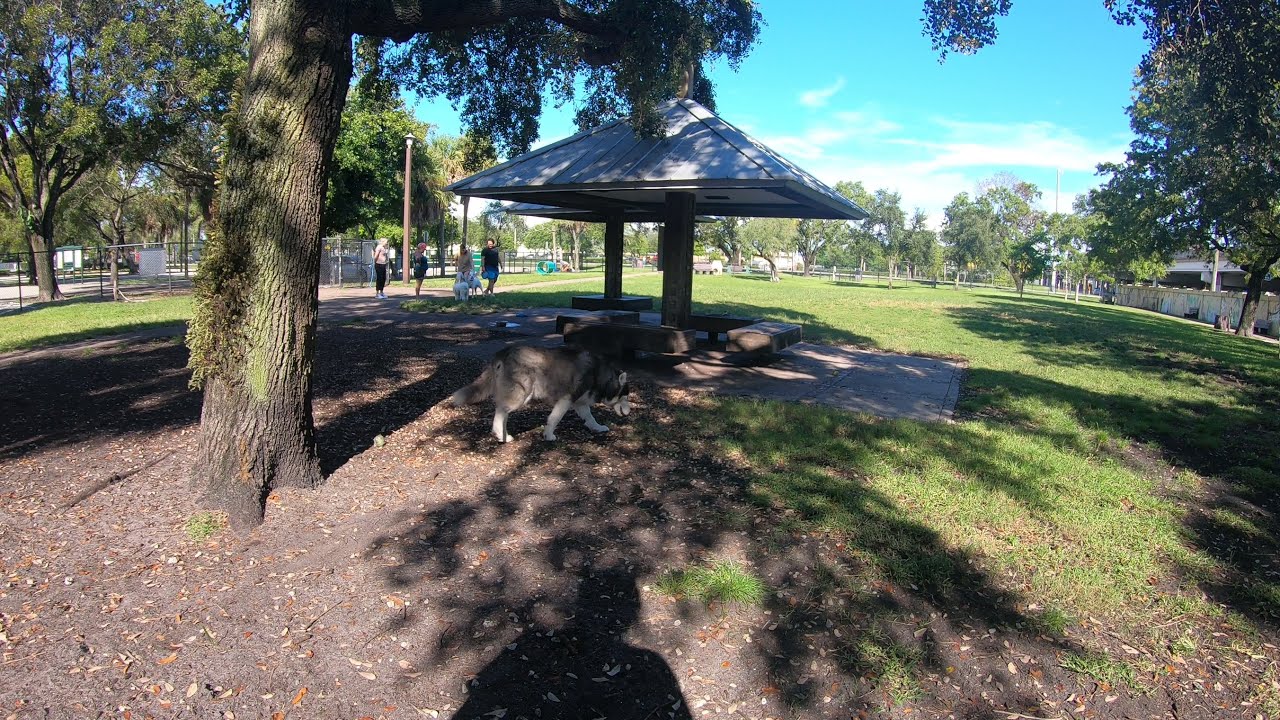In this vibrant daytime scene set in a bustling public park, the focal point is a picturesque kiosk with a distinctive triangular white roof, situated at the center of the image. Directly in front of the kiosk stands a majestic, large tree, its leafy branches casting intricate shadows on the grassy ground. Beneath the tree, a dog with a brown body and four white legs stands, adding life to the serene setting. This dog seems unattached to a leash and is possibly heading towards the kiosk. To the left and right of this central setup, several people are strolling through the park, including three women and a man seen in the background to the left, accompanied by two white dogs of different breeds. Scattered around the kiosk are tables and seating areas, providing a spot for park visitors to rest and seek shade. The clear blue sky above is dotted with white clouds, enhancing the pleasant ambiance. Encircling the park are numerous trees, their shadows stretching across the grass, contributing to the overall cool and tranquil environment. In the rear of the image, dog play structures such as tunnels can be spotted, suggesting this area might serve as a dog park. The image exudes a laid-back, inviting atmosphere of a sunny day perfect for a leisurely outing.